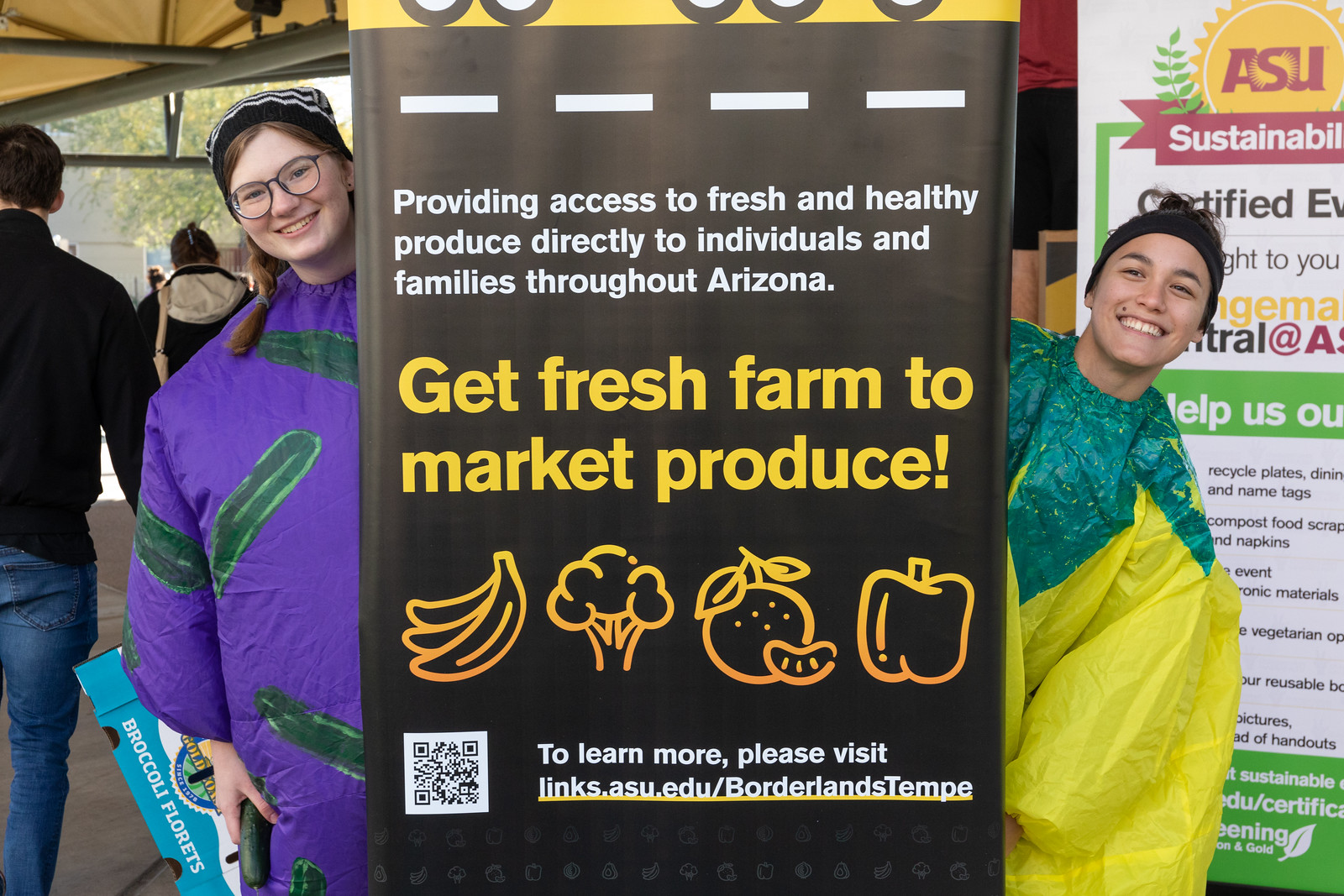In a vibrant and playful scene, two individuals pose behind a large, visually striking sign at a produce market. The sign is a deep black with a blend of white and yellow text. At the top, in white letters, it reads, "Providing access to fresh and healthy produce directly to individuals and families throughout Arizona." Beneath that, in bold yellow text, it declares, "Get fresh farm-to-market produce." The bottom section of the sign features colorful illustrations of various fruits and vegetables like bananas, cauliflower, apples, and peppers, along with text urging visitors to learn more by visiting specific links, accompanied by a QR code.

Peeking out from behind the sign, on the left, is a cheerful young woman with brown braided hair, black glasses, and a black beanie hat. She is dressed in a bold purple jacket festooned with green oval patches resembling cucumbers or pickles. Her outfit's whimsical design, featuring the patches oriented in various directions, adds to the lively atmosphere. Only her smiling face and part of her outfit are visible as she leans out from behind the sign.

Standing on the right is another smiling individual clad in a strikingly oversized yellow windsuit with a green upper section resembling a stem, giving the ensemble a unique, plant-like appearance. This person also wears a black headband and is partially obscured by the sign.

The scene is set under a yellow canopy with black trim, and in the background, several people can be seen, some with their backs to the camera wearing black shirts and hoodies. An ASU Sustainability sign with the words "ASU" in red letters and "Sustainability" in white letters on a red banner is also visible behind them, along with a tree adding to the ambiance of the colorful market setting.